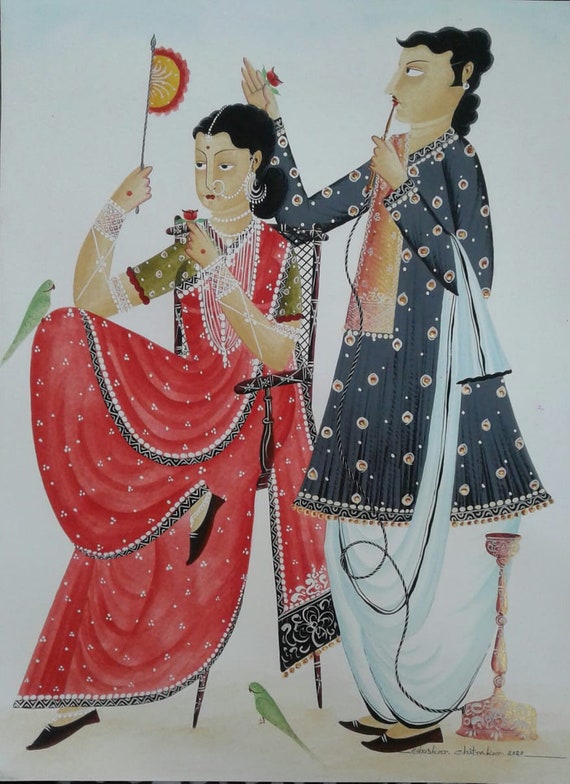This illustration depicts two women of South Asian descent, presumably Indian or Pakistani, dressed in traditional attire. The woman on the left is seated in a high-back chair adorned with a white print. She is wearing a vibrant red sari with a subtle white triangular dot pattern and black trim. Her black hair is pulled back into a bun, and she has medium tan skin. Adorned with a white chain connecting her nose ring to a dangling earring and another chain that extends over her forehead, she also wears a pearl-like white choker and intricate chain jewelry extending down towards her waist. Her right leg is elegantly crossed over her left, and a small green parakeet gently perches on her right knee. She is also holding a small flag, which is red and gold with white stripes.

Adjacent to her, the woman on the right stands gracefully, dressed in a long navy-blue kameez with an intricate peach and white circular pattern and white balloon pants. She also wears a coordinated scarf draped over her right shoulder and black shoes. Her black hair is more relaxed compared to the seated woman, and she shares similar medium tan skin. With her hand, she is delicately placing a small red flower into the seated woman's hair. She holds a gold-colored hookah pipe to her mouth and has a rose in her left hand. A second green parakeet is visible on the floor between the two women. 

The entire scene is set against a void white background, isolating the figures in an elegant, detailed depiction that celebrates traditional South Asian culture. The artist's signature is present but illegible, adding a final mark of authenticity to this detailed artwork.